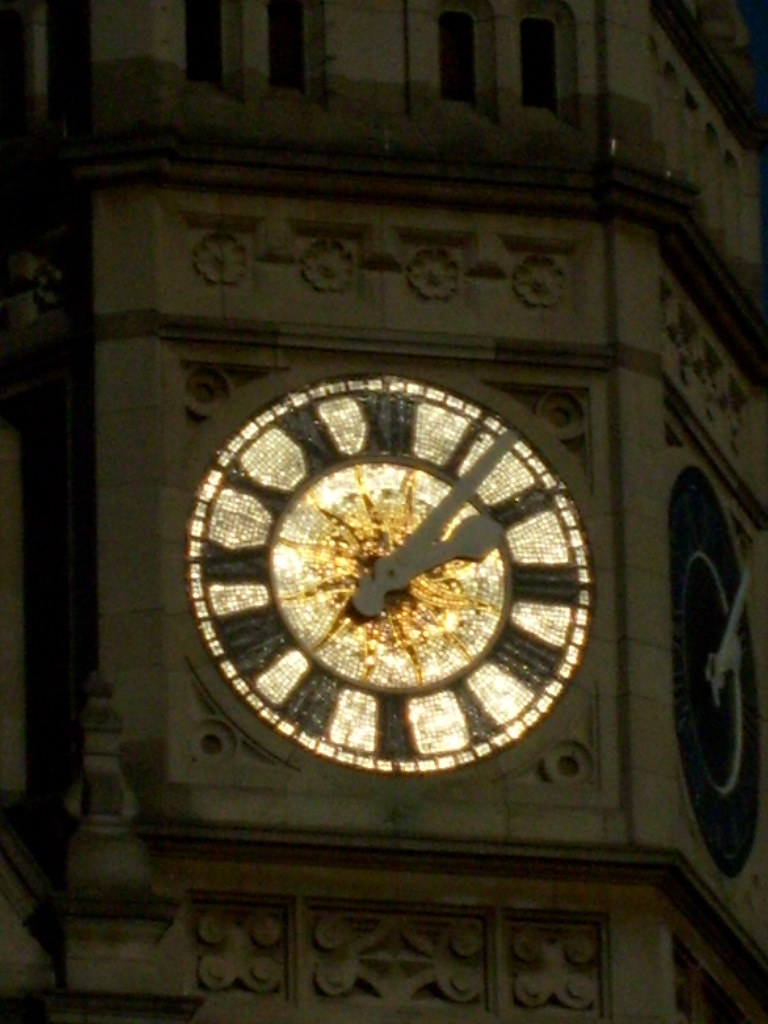The photograph captures an old stone clock tower, shrouded in darkness with only minimal details visible. The image—a vertical, slightly rectangular shot looking upwards at an angle—focuses primarily on the illuminated clock face at the center of the structure. The building itself appears to be made of gray stone, featuring intricate gothic carvings around the clock. The clock face is brightly lit, possibly by a projection, creating a striking contrast against the surrounding shadows. The clock, encrusted with a golden hue, displays Roman numerals, and the time reads approximately 2:06 or 2:07. The large, chunky iron hands—one big and one small—stand out prominently. A second clock face is visible on the far side, but it remains obscured in the darkness, adding a sense of mystery to the scene.